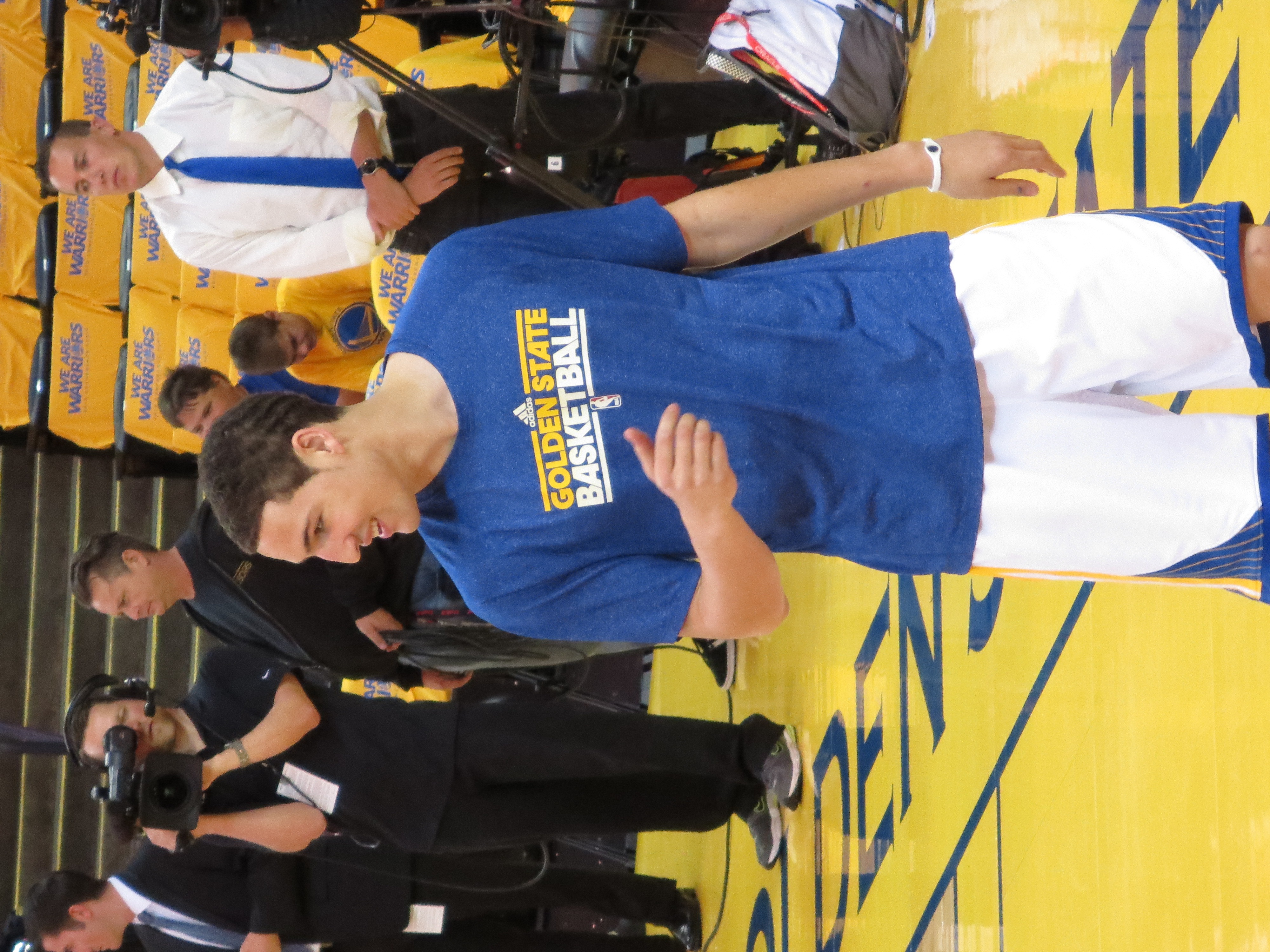This is an indoor photograph of a basketball player standing on a yellow ground with blue text. The player is wearing a blue t-shirt that reads "Golden State Basketball" with an Adidas logo above in yellow. He has white shorts adorned with blue triangular patterns, yellow pinstripes, and additional yellow and white stripes on the sides. The player's left wrist features a wristband or jewelry. The image is tilted 90 degrees counterclockwise, but if adjusted, he would be facing left. Behind the player, a cameraman in black, two individuals in black suits, and a person in a white long sleeve shirt with a blue tie are visible. The setting appears to be a high school or college basketball auditorium, with several other people in black uniforms and yellow-covered seats matching the team's colors.